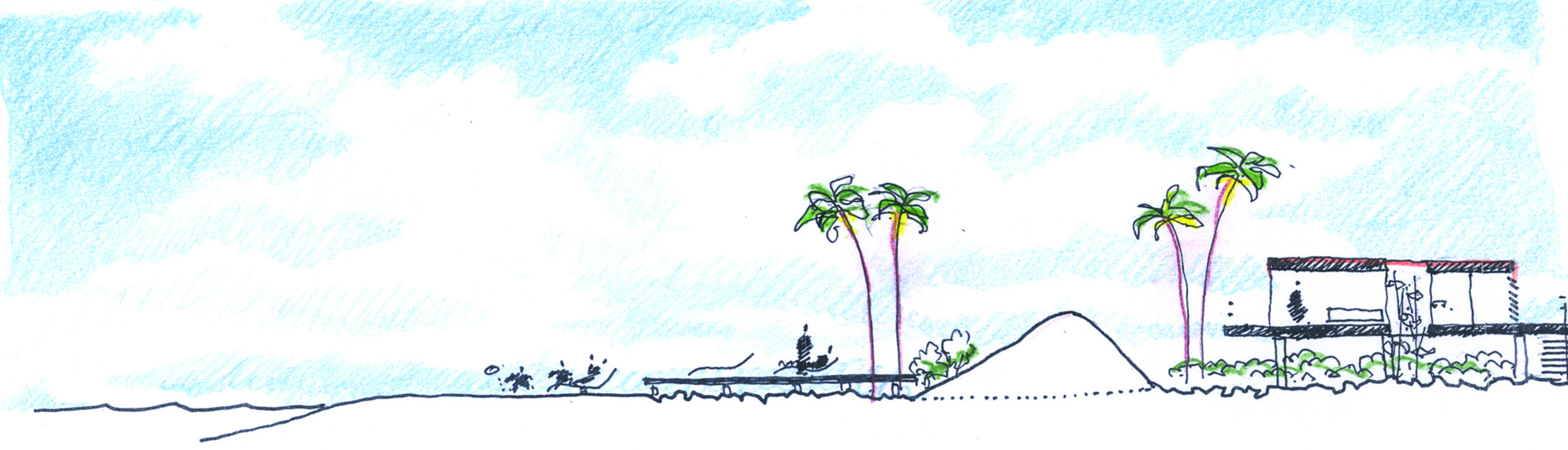This detailed illustrated image, set in a long rectangular frame, depicts a pristine beach scene dominated by striking green palm trees, which stand out vividly against the predominantly black-and-white ink composition. The sky is rendered in a light blue shade with fluffy white clouds scattered throughout, enhancing the serene atmosphere. The beach itself is drawn with white sand and stretches out to the left, where the water begins. In the very center, a wooden pier extends into the ocean, and atop the pier lies a solitary figure, silhouetted and reclining on a chair. To the left of the pier, another silhouette is discernible, seated on a chair by the beach. Nearby, two more indistinct figures, appearing like playful blobs, might be engaged in a game, with one seemingly tossing a ball.

A white hill divides the scene, cresting in the center and flanked by two clusters of lush, bushy palm trees on either side—two on the left and two on the right. On the far right side of the image, a modern-designed house or building rises on posts above the ground. A figure is just barely visible within this elevated structure, adding a sense of human presence to the tranquil setting. The overall composition is a harmonious blend of nature and subtle human activity, capturing the essence of a peaceful day by the beach.